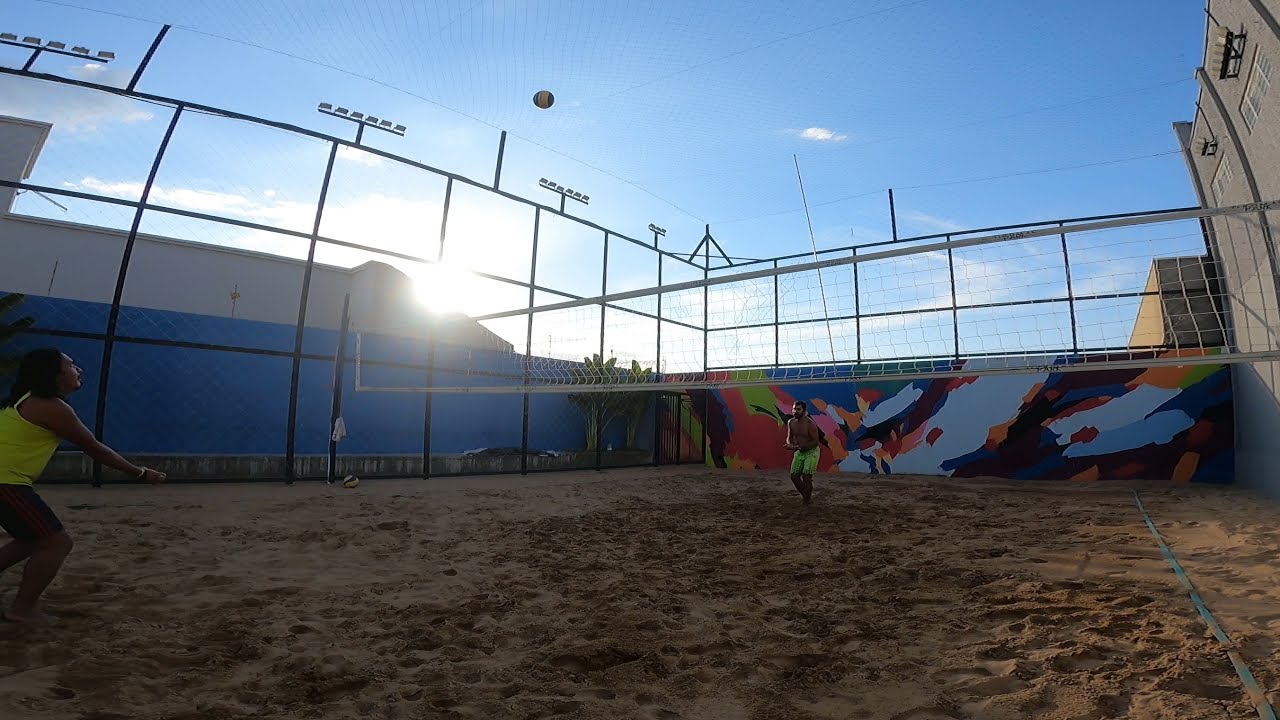In this detailed photograph of an outdoor, beach-style volleyball court, two players are engaged in a lively match under a bright, sunny sky. The court, filled with sandy ground bearing numerous footprints, is enclosed by high walls and exceptionally tall fencing, giving it a somewhat urban feel. The bright sun peeks over a gray building to the left, casting light across the mid-day scene. On the left side of the court stands a player wearing a yellow tank top and dark shorts, preparing for action. Opposite him, a bare-chested player in green shorts is poised on the right. The volleyball, captured midair, hovers just above the net, centrally positioned. High-rise buildings frame the scene on both sides, accentuating the court's urban setting. The sky above is a vivid blue, dotted with a few white clouds, completing this vibrant snapshot of a sunny-day volleyball game. The colors in the image include shades of yellow, brown, black, tan, lime green, light blue, orange, white, blue, red, and maroon, adding depth and vibrancy to the composition.